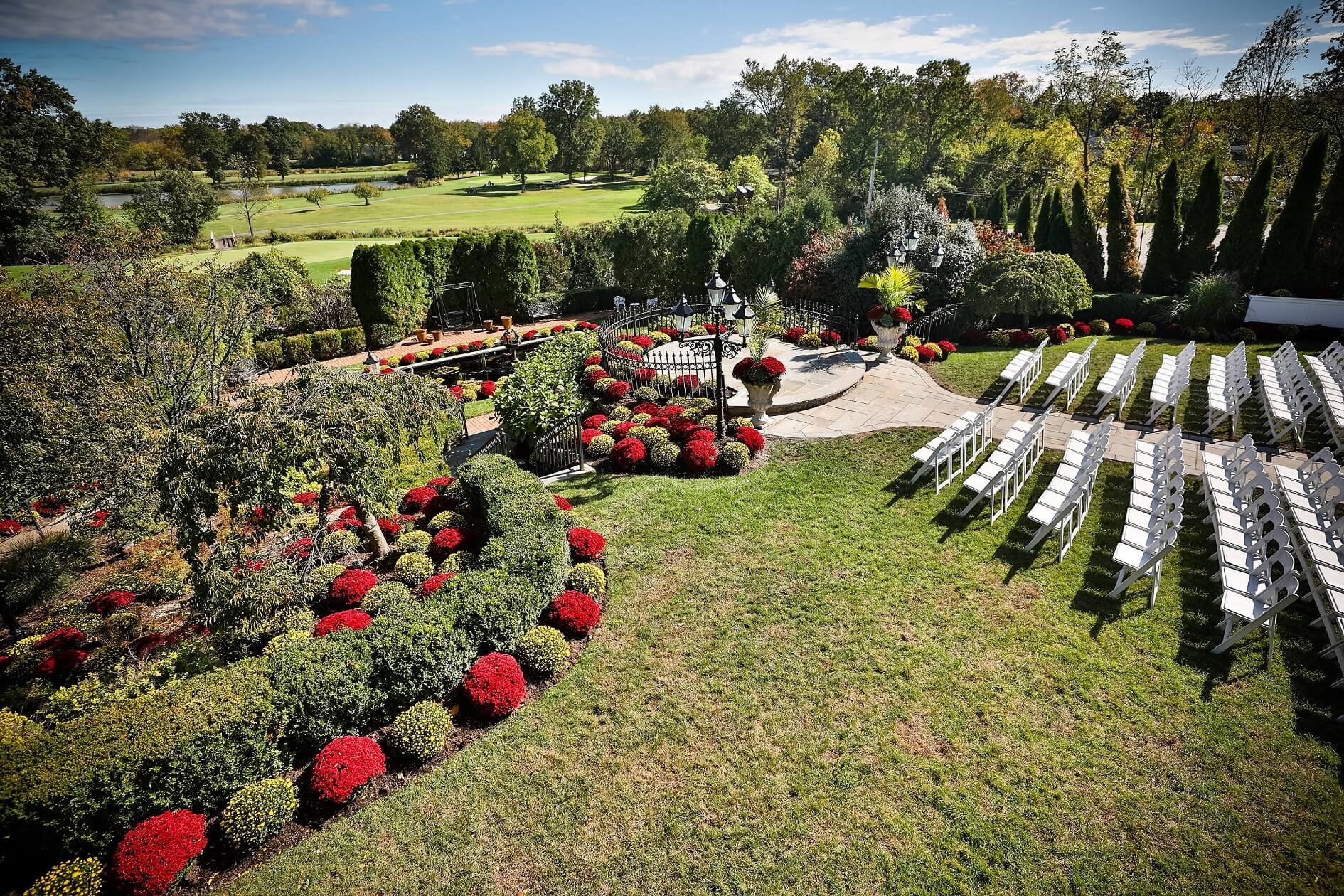This photograph, taken from an elevated, bird's-eye view, captures a beautifully manicured public garden set up for a wedding ceremony. The central focus is a small cement platform surrounded by a black iron fence, positioned in the middle right of the frame. A cement pathway leads up to this platform, flanked by rows of white folding chairs neatly arranged on either side of the walkway. The garden itself features a variety of well-maintained shrubs, with a mix of vibrant green and bright reddish hues, adding a picturesque contrast. To the left of the image, the background extends into a rolling grassy area that resembles a golf course, complete with a serene pond and tall green trees that enhance privacy. The sunny day illuminates the entire setting, highlighting the lush greenery and the tranquil ambiance, though no people are present in the image.